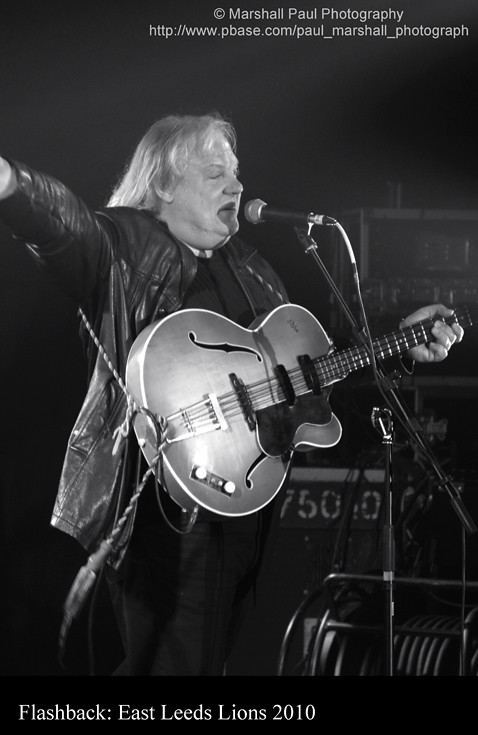This black and white photograph, credited to Marshall Paul Photography, captures a moment from the Flashback East Leeds Lions 2010 event. The scene shows a male musician, identifiable by his long blonde hair and heavyset appearance, in mid-performance on stage. He is dressed in a black outfit, consisting of a leather jacket, shirt, and pants, and is positioned against a dark, indeterminate background. The man is holding a guitar, which is strapped across his body, and sings into a microphone that's mounted on a stand. His left hand grips the neck of the guitar, while his right arm is extended out to the side, pointing slightly off-frame. The photo features a black border at the top and bottom, with the text "Flashback East Leeds Lions 2010" and the copyright information for Marshall Paul Photography, including the web address, printed below the image.